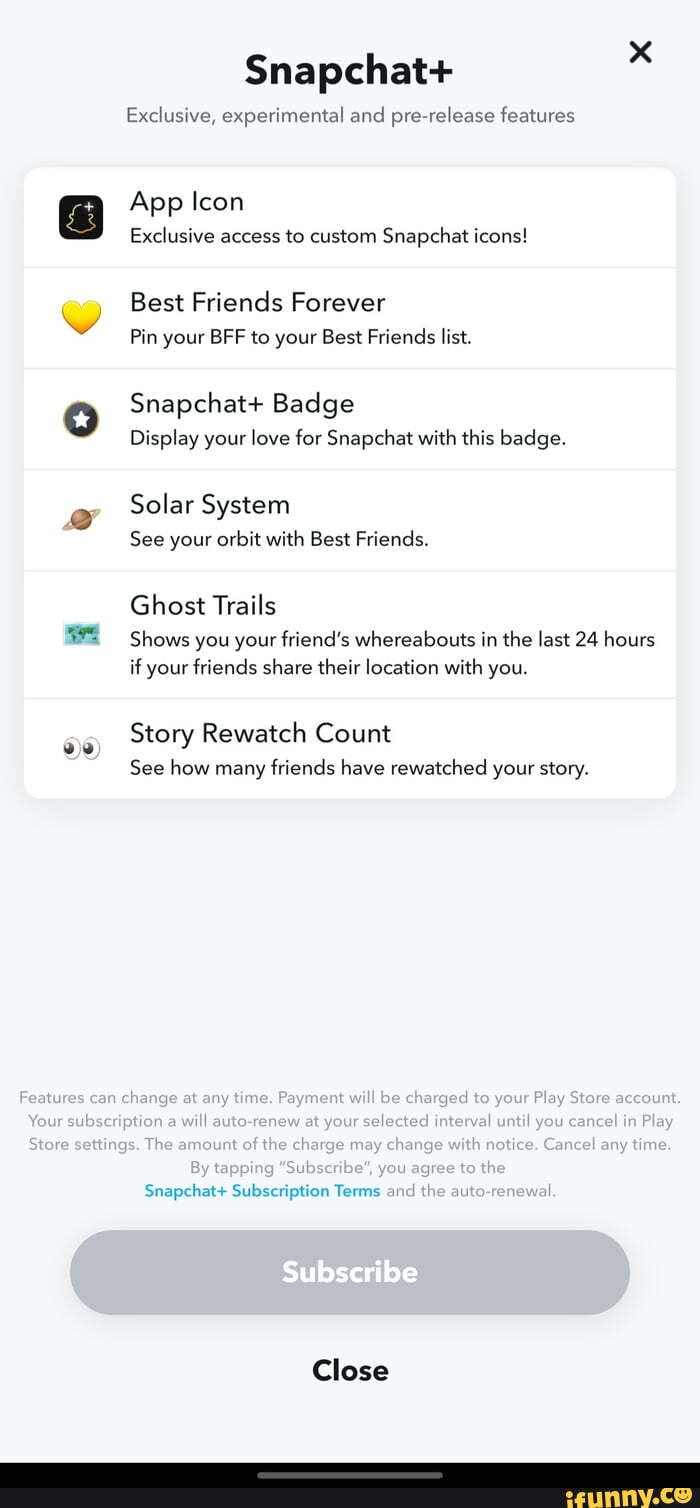The image showcases a Snapchat screen on a mobile phone. The screen has a light blue background. At the top, the title "Snapchat Plus" is prominently displayed in dark black text, with a small "X" in the upper right-hand corner for closing the screen.

Beneath the title, a description reads: "Exclusive, experimental, and pre-release features." Below this description, there is a white box divided into six distinct strips, each detailing a different Snapchat Plus feature:

1. **App Icon**: The first strip features an image of a black square with a bell icon inside it. The caption reads "Exclusive access to custom Snapchat icons."

2. **Best Friends Forever**: This section is symbolized by a yellow heart. The accompanying text states, "Pin your BFF to your best friends list."

3. **Snapchat Plus Badge**: Displayed with a black circle containing a white star, this strip says, "Display your love for Snapchat with this badge."

4. **Solar System**: Represented by a planet with a ring around it, the text explains, "See your orbit with best friends."

5. **Ghost Trails**: Shown with a greenish box, this feature allows you to "Show your friends' whereabouts in the last 24 hours (when friends share their location with you)."

6. **Story Watch Count**: Illustrated by two eyeballs, this option lets you "See how many friends have re-watched your story."

At the bottom of the screen, there are two buttons: a gray "Subscribe" button and another for closing the page.